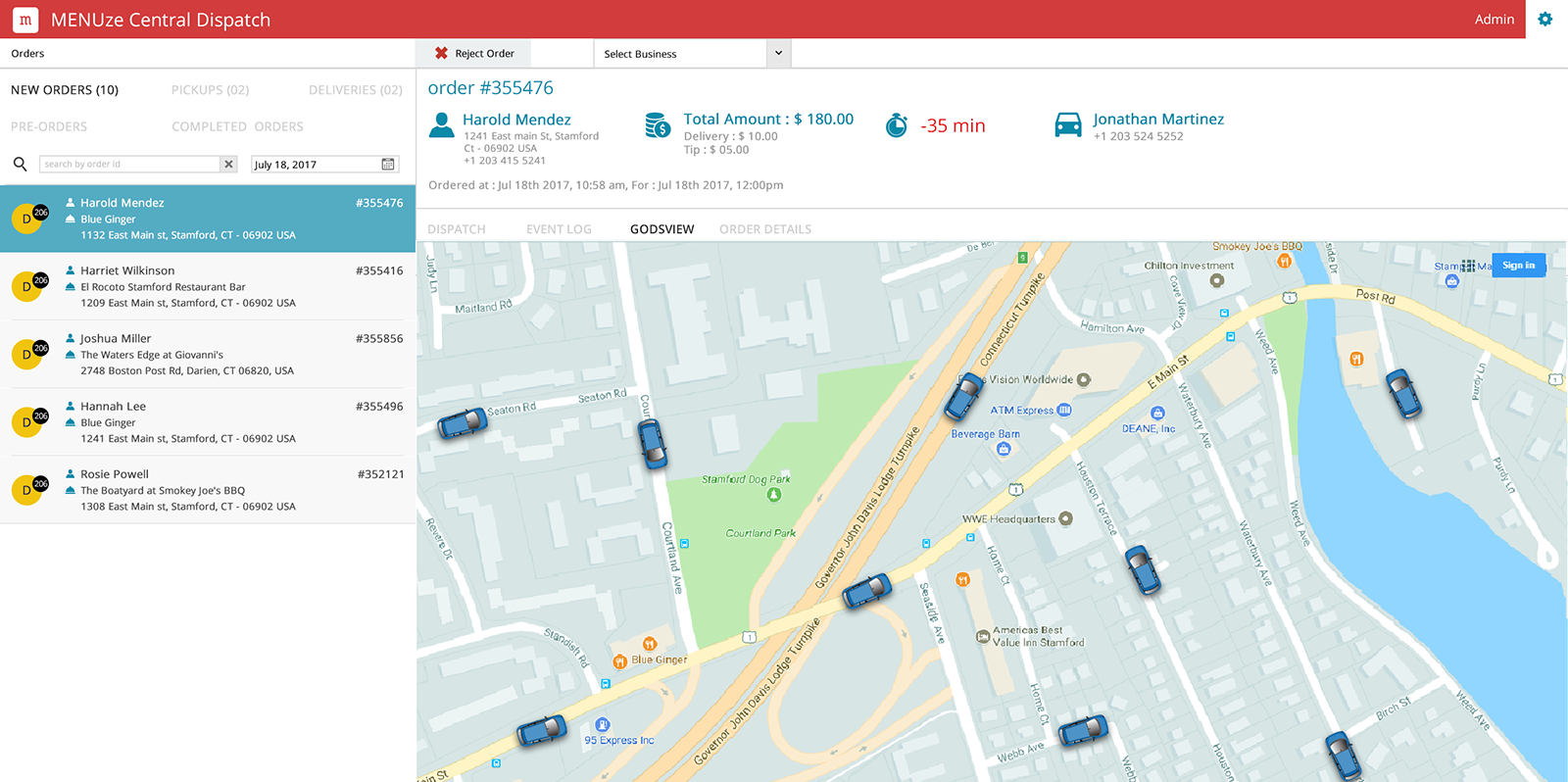This image depicts a web interface for a platform named "MENUZE", where "MENU" is emphasized in capital letters and "ze" in lowercase. In the upper left corner of the screen, there is a white square containing text that is too indistinct to read. Adjacent to this square, "Central Dispatch" is prominently displayed in a red banner at the top of the page. On the upper right corner, there is the label "Admin" accompanied by a cogwheel icon, suggesting configuration or settings options.

Below the banner, the left side of the interface features a vertically aligned menu. At the top of this menu, the word “Orders” is aligned to the left. Directly underneath, “New Orders” is listed with the number “(10)” in parentheses next to it, indicating ten new orders. A couple of additional category labels, likely “Pickups” and “Deliveries,” are partially visible but hard to discern due to distance and faded text. Further down, categories titled “Pre-orders” and “Completed Orders” are also present, each accompanied by rectangular boxes.

In the main body of the interface, five rows can be seen, each beginning with an overlapping double-circle icon containing the letter "D". Each row includes two lines of information and ends with numeric values. For example, the middle row features:

- Order Number: 355476
- Customer Name: Harold Mendez, followed by an icon
- Total Amount: $180
- Time Indicator: -35 minutes
- Delivery Agent: Jonathan Martinez with a car icon

The lower section of the screen seems to include a map with car icons, possibly indicating delivery routes or real-time tracking of orders.